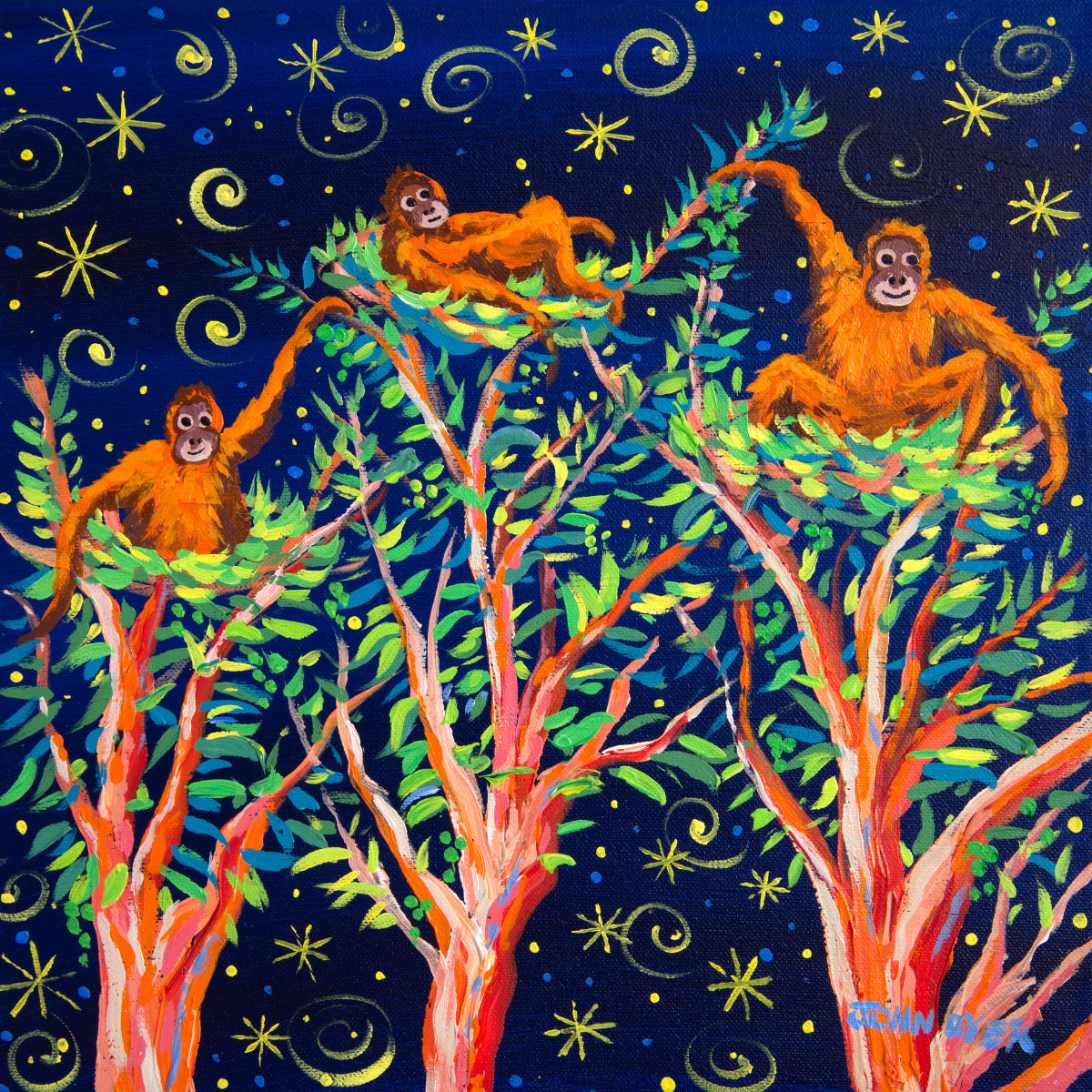This vividly colored acrylic painting depicts three animated orangutans each positioned atop a tall tree adorned with an abundance of individually painted green leaves in various shades. The tree trunks exhibit reddish-brown hues accented by lighter white strokes. The central orangutan is reclining on the tree's upper branches, while the two flanking orangutans are seated, each extending an arm to touch a branch of the middle tree. The background is an imaginative starry night consisting of numerous blue and yellow dots representing stars, larger star shapes, and abundant yellow swirls scattered throughout the dark blue gradient sky. The piece is signed by the artist, "John," although the last name is indecipherable, and the signature is located in the bottom right corner. The painting is rich in detail and animated in style, creating a vibrant and lively scene.